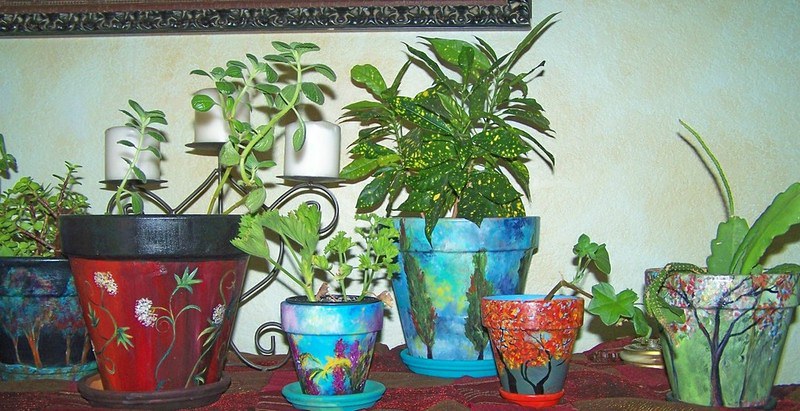The image depicts a horizontally oriented painting, approximately two and a half times wider than it is tall, showcasing a series of six vividly painted flower pots, each containing different types of green plants without blooms. The pots rest on a table draped in what appears to be a red tablecloth, possibly with some fabric texture. Behind the arrangement is a light blue, splotchy wall with the bottom edge of a black and silver picture frame visible. 

From left to right, the arrangement begins with a large blue pot brimming with green plants characterized by slender brown stems and small leaves. Next is a red flower pot with a black rim, painted with delicate white flowers. The third pot is blue with an aquatic scene featuring fish on the side, followed by another blue pot adorned with images of tall, thin trees with green leaves. The fifth pot, painted red with a depiction of autumnal trees bearing red and yellow leaves, holds a somewhat bent green plant. The final pot is green, displaying a tree with red leaves, and houses a leafy green plant speckled with yellow. Sitting behind the largest pot—a bright red one on the left—is a wrought iron candelabra supporting three large candles. The plants range in height from three to ten inches and include varieties from succulents to leafy types.